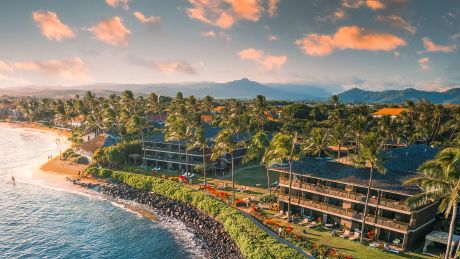The image depicts a scenic coastal resort area, possibly in Hawaii. The setting features multiple three-story hotel or condo buildings, two of which are prominently placed—one in the bottom right-hand corner and the other in the middle of the image. The foreground of these structures is lined with lounge chairs on the patios. The resort is nestled against a rocky coastline with a small stretch of beach on the left-hand side, where small waves meet the shore. The ocean, taking up the bottom left-hand corner, contrasts beautifully with the abundant greenery. Palm trees are scattered throughout the scene along with various other foliage and patches of red plants.

In the background, a majestic mountain landscape rises, creating a dramatic contrast with the serene blue ocean. Smaller homes are visible further up the coast, suggesting a blend of private and commercial properties. The sky is partly cloudy, adding depth to the visual composition, and the light in the scene hints that it could be nearing sunset. The vivid color palette includes deep blues, whites, various shades of green, reds, grays, browns, blacks, and oranges, providing a rich and vibrant atmosphere to the resort area. There are no people visible in this picturesque and peaceful snapshot.